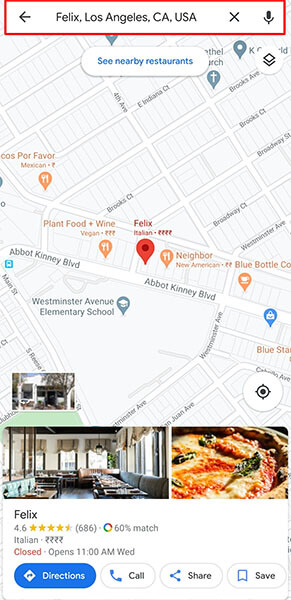This detailed map highlights various points of interest in the Felix neighborhood of Los Angeles, California, USA. Several markers indicate nearby restaurants, including "Plant Food and Wine," "Tacos Por Favor," "Neighbor," "Blue Bottle Coffee," and "Felix." There is also a marker for a church and another for Westminster Avenue Elementary School, located at the intersection of Bikini Boulevard. 

The map prominently features a section at the bottom devoted to Felix, a highly-rated Italian restaurant with a rating of 4.6 stars. Although currently closed, it is set to open at 11 a.m. on Wednesday. The listing includes buttons for getting directions, making a call, sharing the location, and saving it for future reference.

An inset photograph reveals the restaurant's interior, showcasing a long dining area with booth seating along both walls. Each booth is accompanied by tables with additional chairs on the opposite side, forming a central aisle lined with chairs. The back right-hand corner features a cozy circular booth. The restaurant’s design is further enhanced by large front and side windows, which allow ample natural light to flood the space.